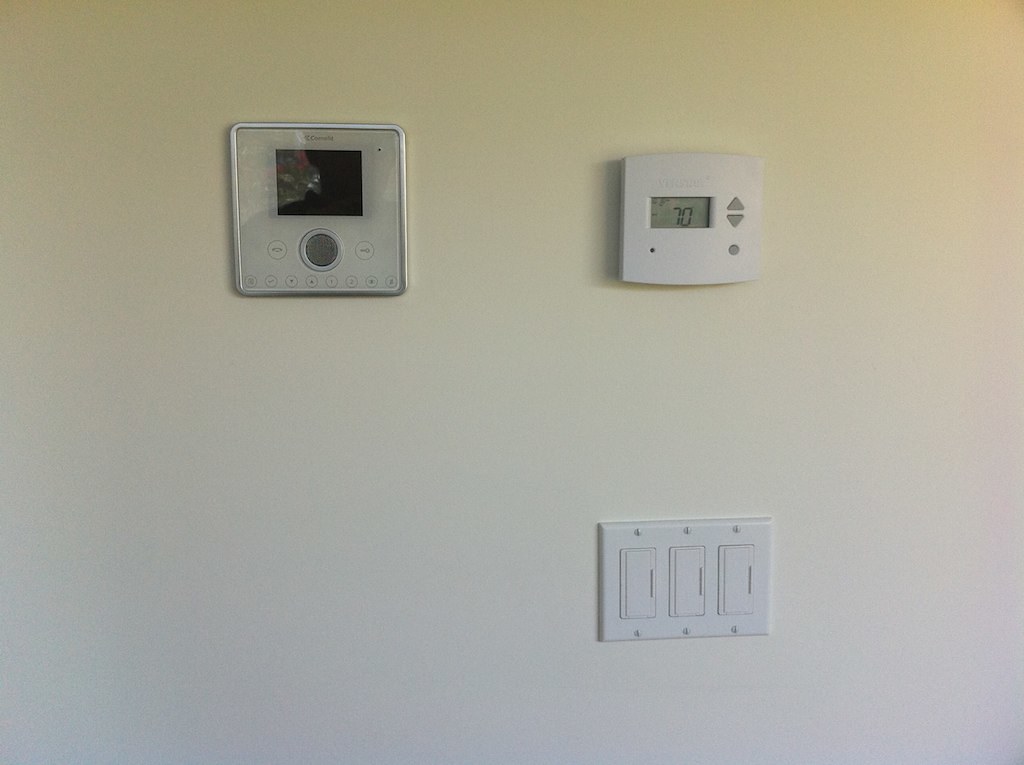The image depicts a white wall background with two distinct devices and three switches prominently featured. In the top left corner, there is a device with a plastic cover. The device has the word "brand" at the top and features three central buttons: a large grey middle button flanked by a button on the left and a button on the right. Below these, eight additional buttons are evenly spaced along the bottom edge of the device.

Adjacent to the device on the right, there is a white thermostat. The thermostat display reads "70" with some text at the top. To the right of the display, there are three controls: an upper grey arrow, a lower grey arrow, and a grey button.

In the lower section of the image, three square push switches with visible screws at the top and bottom are seen. Each switch includes a small protruding bar. These switches appear to be off, though there is a slight illumination noticeable at the lower end of the image, suggesting some form of backlight might be present.